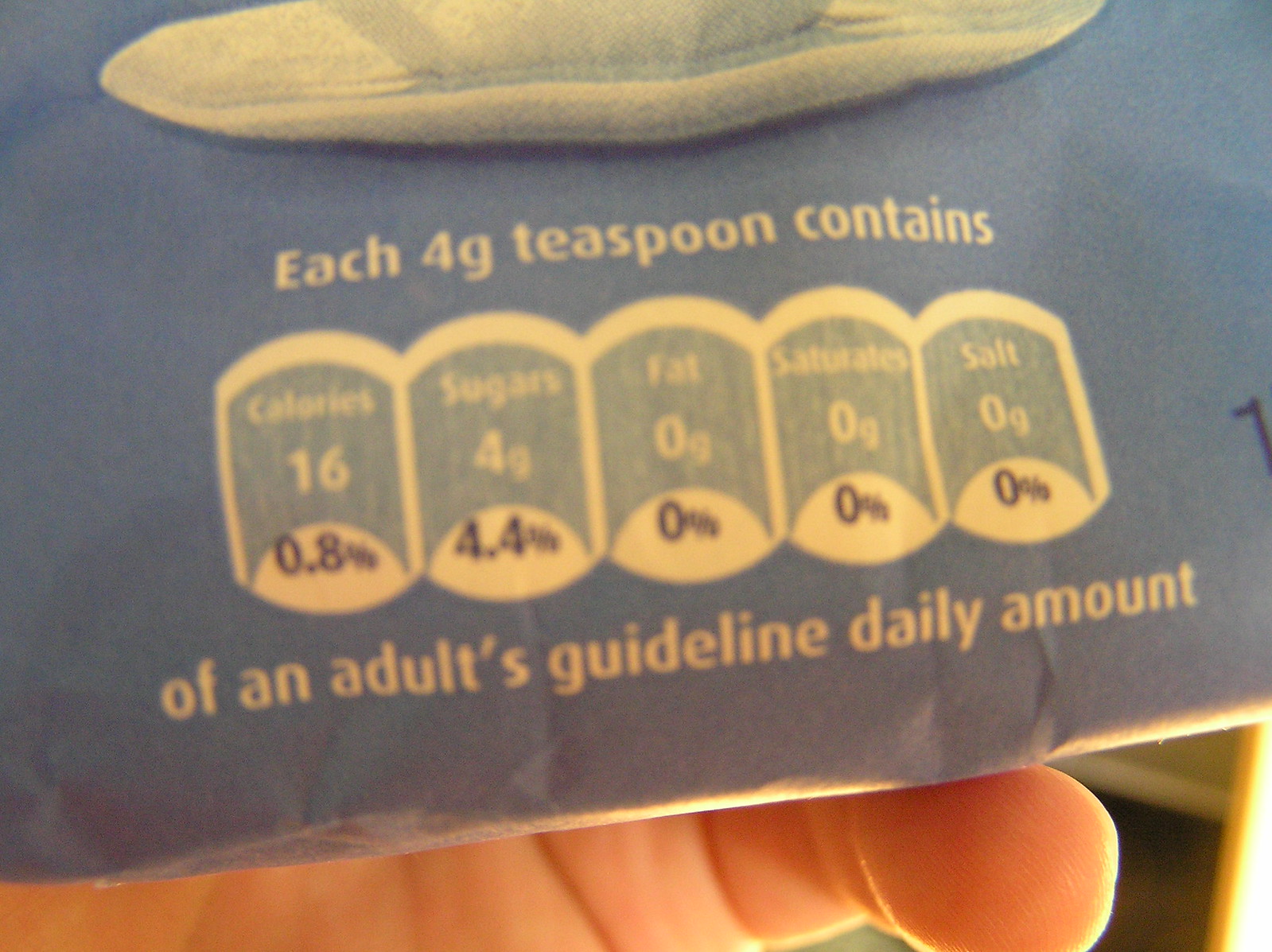This photograph captures the nutritional information on the blue rear side of a food package, likely a sugar packet, showing a close-up of ingredients summary. The text on the packaging, in a light brown or cream color, clearly states that each 4-gram teaspoon contains 16 calories, 4 grams of sugar, 0 grams of fat, 0 grams of saturates, and 0 grams of salt, which aligns with an adult's guideline daily amount. The image is rectangular and also features part of a person's finger holding up the package, adding a touch of human interaction to the detailed nutritional breakdown.